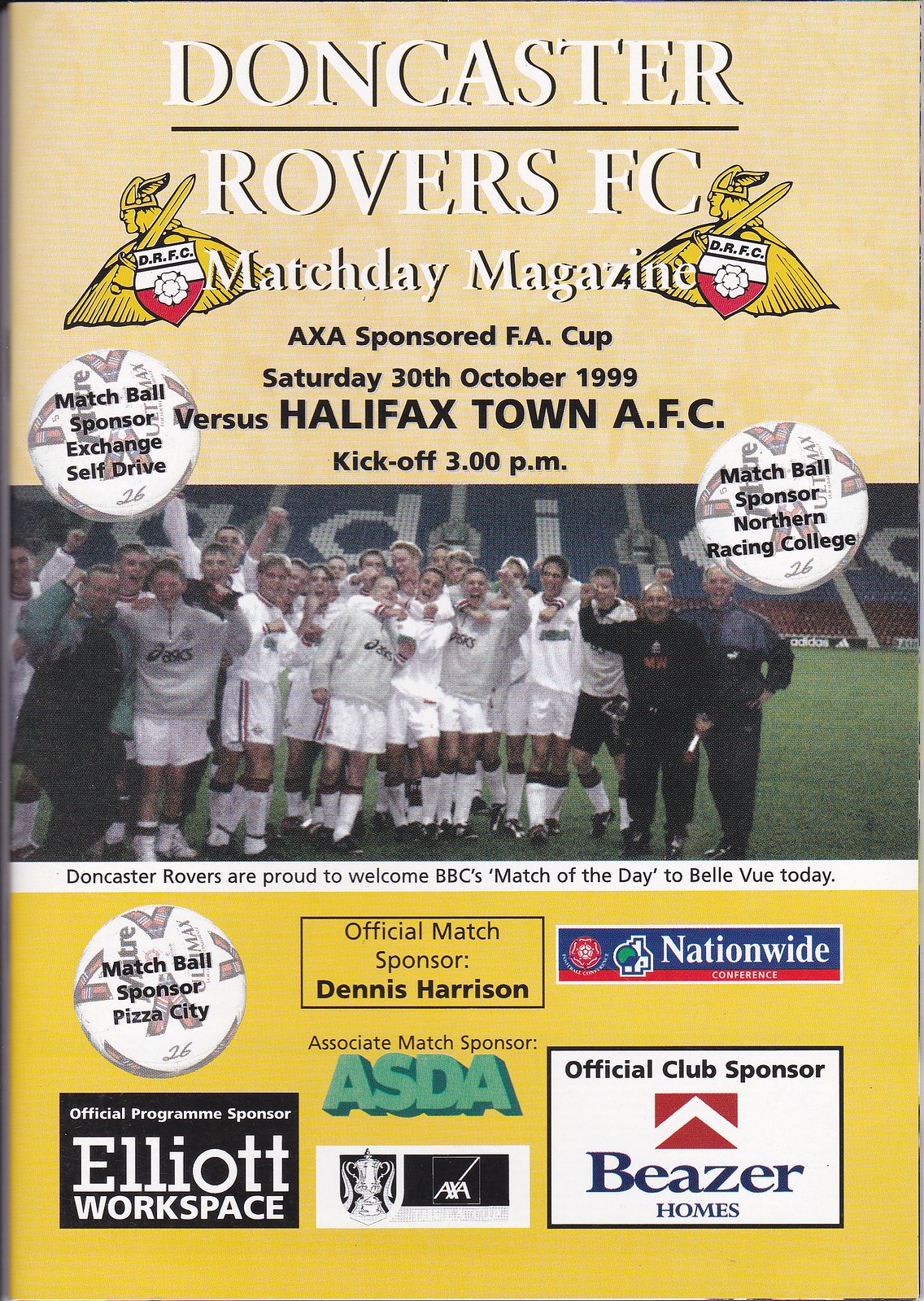This detailed magazine cover of the Doncaster Rovers Football Club's match day program for October 30th, 1999, predominantly features yellow and beige hues. The top of the cover announces the match between Doncaster Rovers and Halifax Town AFC, with kickoff at 3 p.m., and highlights AXA as the FA Cup sponsor. Central to the cover is a photograph of the jubilant Doncaster Rovers team, clad in white uniforms featuring the ASICS logo and various sponsor insignias, seen hugging and raising their hands triumphantly. The bottom section of the cover lists multiple sponsors, including Pizza City, Elliott Workspace, Beezer Homes, Dennis Harrison, ASDA, Nationwide Conference, and AVA. The caption beneath the team photo reads, "Doncaster Rovers are proud to welcome BBC's Match of the Day to Bellevue today." The image is styled as a vertical rectangle, with sponsor logos neatly arranged at the bottom, effectively highlighting the team’s camaraderie and the event details.